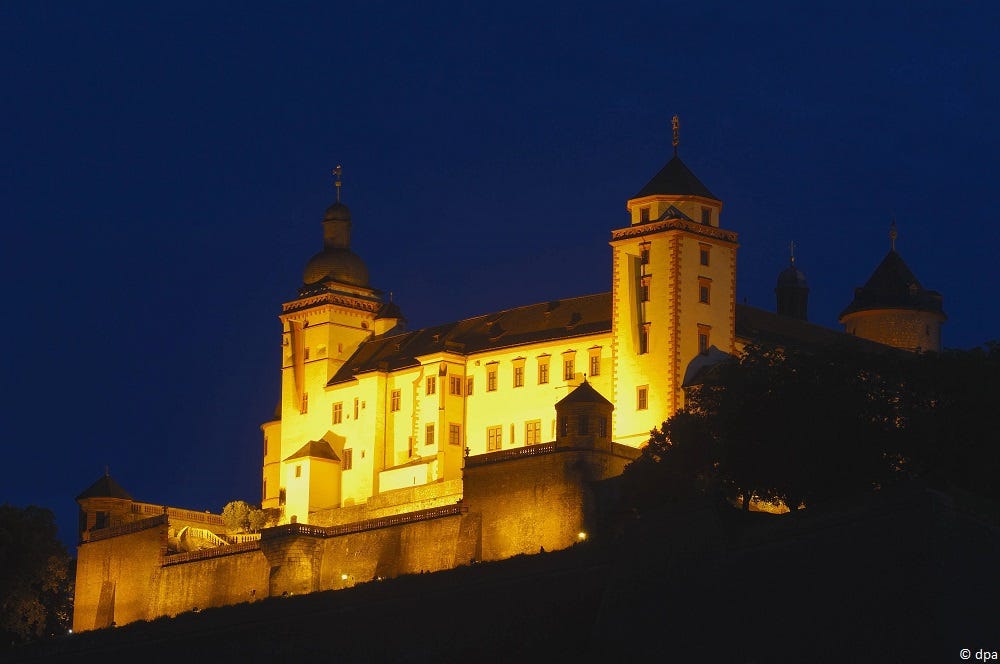In this captivating nighttime photograph, an imposing European castle sits majestically atop a hill, its facade bathed in a warm orange glow that stands out against a deep navy blue sky, free of clouds. The castle is surrounded by a solid concrete wall topped with metal barriers, presumably for security, and features guard towers at each corner. The expansive structure exhibits formidable architecture with two prominent pillars that rise like towers flanking either side of the main building, which itself reaches about three stories high, capped with additional floors in the pillars extending to roughly four stories. 

The building is adorned with many windows—approximately seven horizontally across three rows—allowing glimpses into its grandeur. Darkened forestry lines the base of the hill, with a distinct tree on the bottom left and some shrubs on the bottom right, adding to the secluded and protected aesthetic of the castle grounds. The bottom right corner of the image also contains a faint watermark reading "DPA ©," indicating its proprietary nature. The dim light of early nightfall, coupled with the castle's illumination, creates a striking and enchanting visual display.